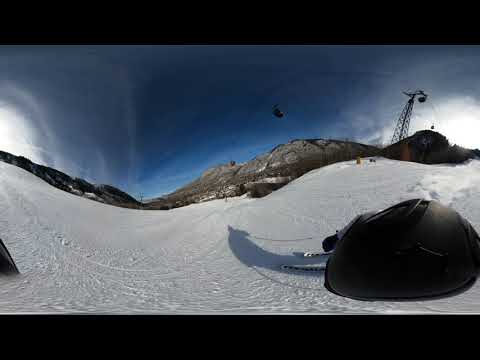The image presents an expansive, wintry landscape at what is likely a ski resort. Taken with a fish-eye lens, the photograph has a distinct distorted effect, enhancing the wide and curved appearance of the scene. The bright blue sky occupies the upper portion of the image, dotted with misty clouds. Jagged rock formations of a mountainous backdrop meet the ground along a sweeping, curved horizon. The snowy terrain stretches out below, heavily marked by ski trails that crisscross the area.

In the sky, a person is captured mid-air, likely having just leaped from a ski jump, adding a dynamic element to the scene. The lower right corner features a black object, possibly a helmet, and its shadow, suggesting the presence of skiers. Additionally, the photo includes infrastructure details such as cable cars on a tower and a large crane, hinting at the resort's operational elements. There might also be a helicopter hovering in the center, indicative of aerial activity common in such high-altitude winter sports environments. The image's black header and footer, which frame the landscape-oriented shot, accentuate its expansive, panoramic quality.